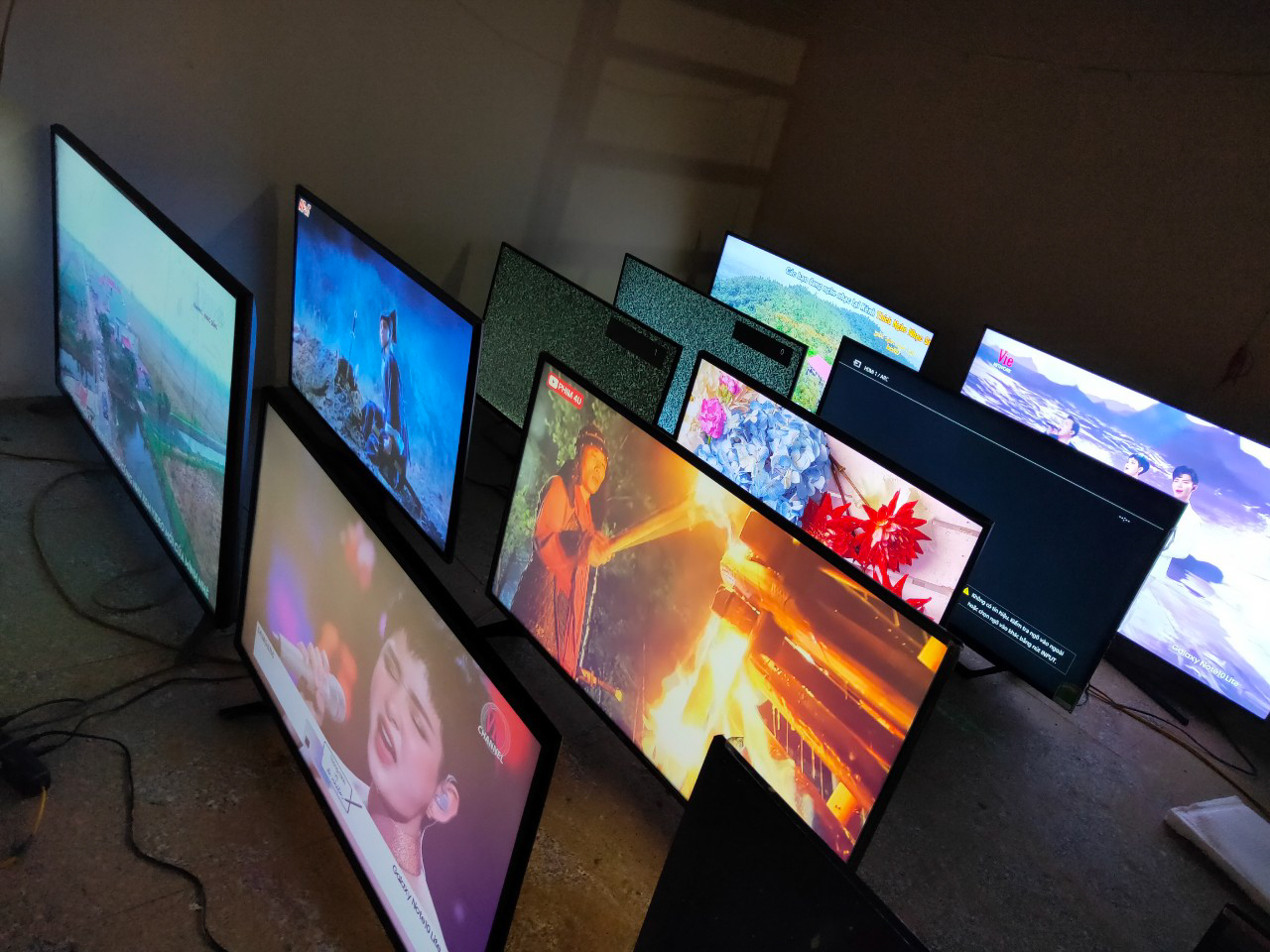The image depicts a dimly lit room with grayish walls and a tile or stone floor. The focal point of the room is a collection of ten large, flat-screen monitors arranged in two diagonal rows of five. Each monitor displays various brightly colored images, ranging from movie scenes to music video clips, cityscapes, and aerial views of geographic locations. One notable screen near the front shows what appears to be a YouTube video of a man involved in glass blowing or pouring molten liquid. Among the different displays, two monitors at the back exhibit green static screens, and one has an error message. The monitors are powered by black cables that trail from the lower left out to each device. A faint shadow of a ladder is visible on the wall, adding to the room’s somewhat industrial and unfinished ambiance.